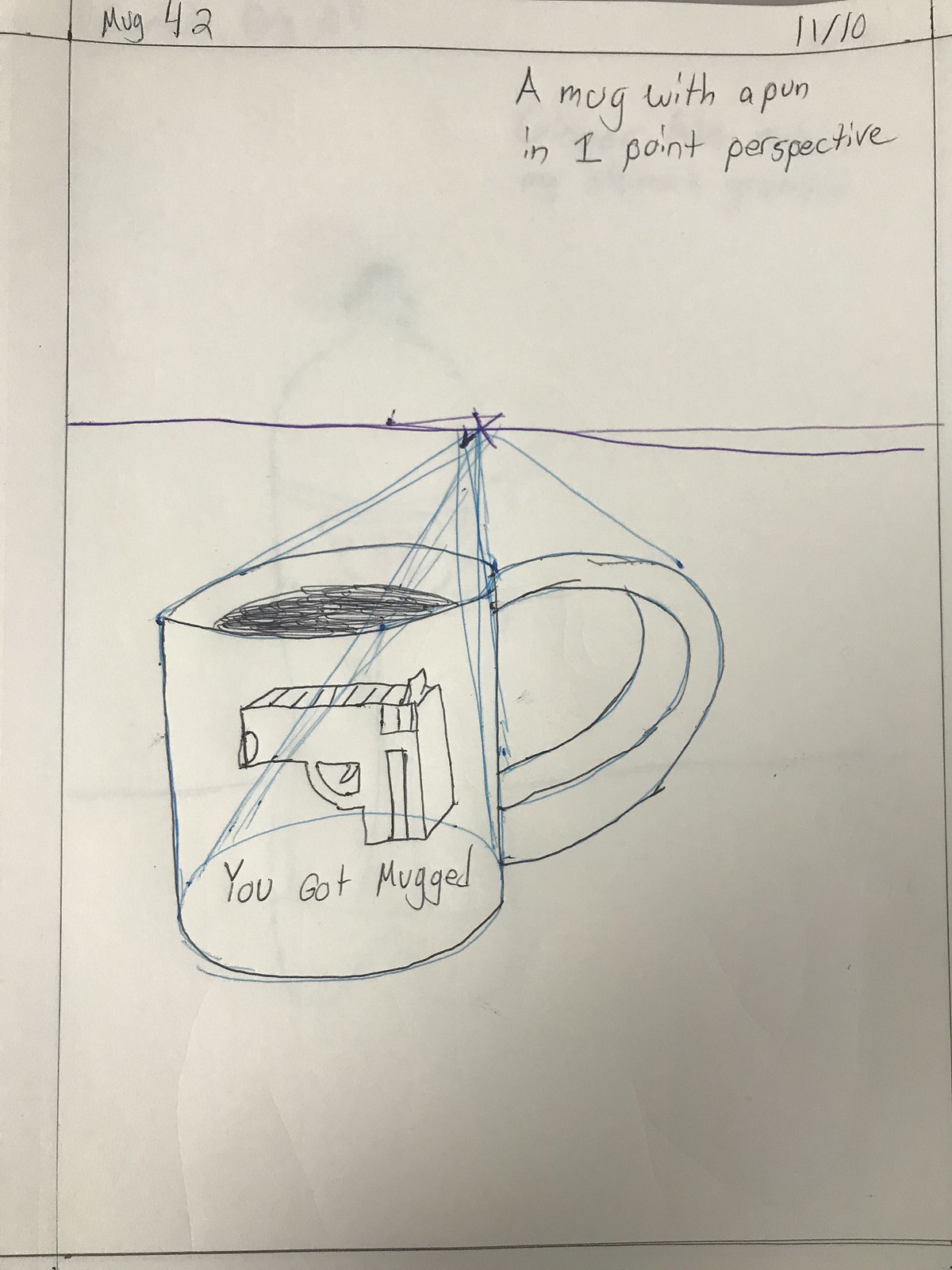The image depicts a detailed pencil and ink drawing on white paper, illustrating a one-point perspective of a coffee mug. At the top left corner, the drawing is labeled "mug 42," and the top right corner contains the numeric annotation "1110." Also in the top right, it's inscribed in black pen, "a mug with a pun in one-point perspective." Below a horizontal purple line that spans the width of the paper, there is a meticulously drawn coffee mug. The mug, outlined in pencil, features black scribbling to simulate being filled with a dark liquid, presumably coffee. On the front face of the mug, a gun's butt and trigger are illustratively rendered, with the phrase "you got mugged" written underneath, adding a humorous pun to the artwork. Lines extending from the mug accentuate the one-point perspective, emphasizing depth and dimensionality.